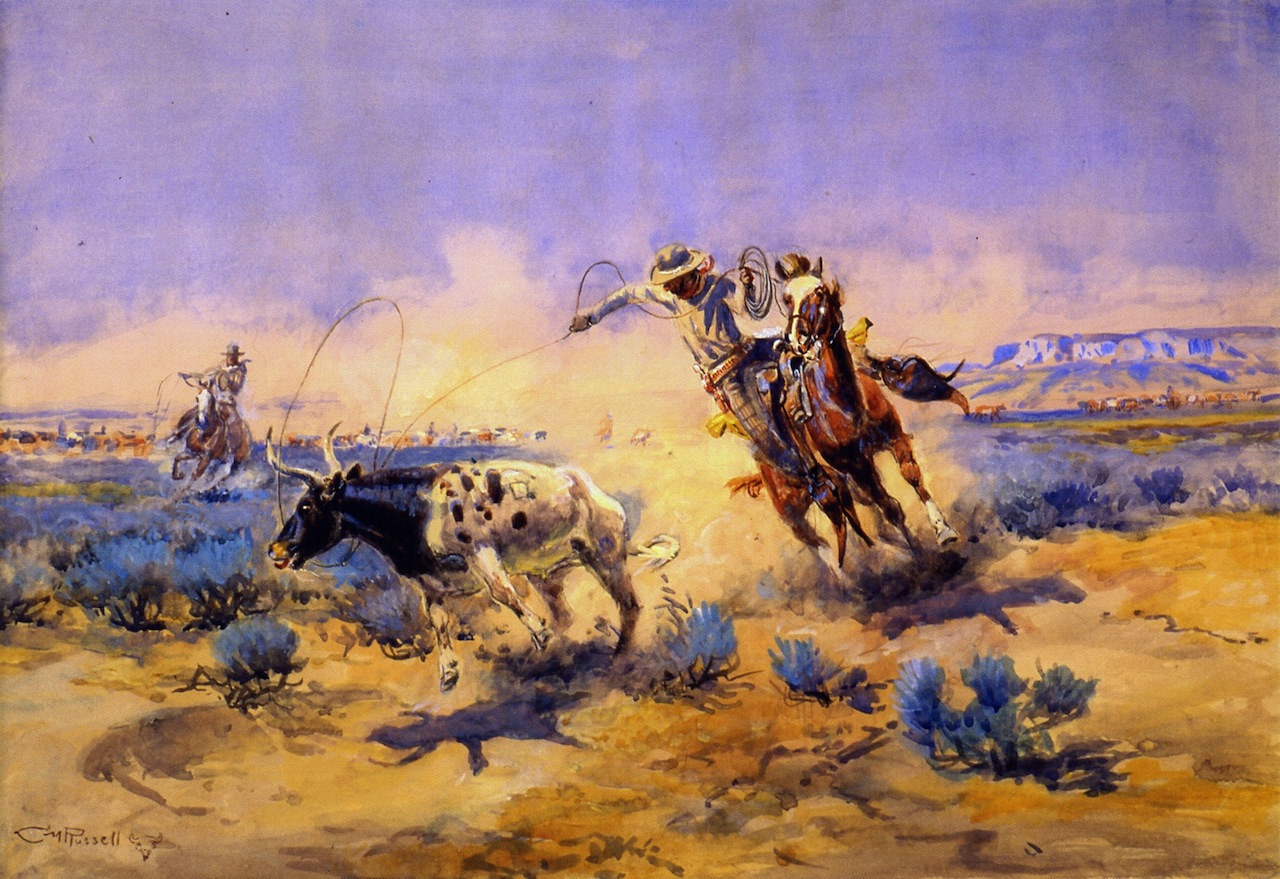This vibrant painting captures a dramatic Wild West scene where two cowboys on horseback are roping a steer in the open desert plains. The steer has a striking appearance with its white body adorned with black speckles, a black head and neck, and a tan snout, along with long white horns about two feet in length. The cowboy in the forefront, riding a brown horse, is skillfully maneuvering to secure his lasso around the steer's head, while another cowboy on a brown horse trails behind with his rope ready, possibly aiming for the steer's hind legs. The ground is a mix of yellow sand and blue bushes, with a purplish sky overhead that adds to the mystique of the scene. In the background, there's a flat-topped mountain and hints of more cattle, underscoring the rugged, expansive landscape characteristic of the western frontier.